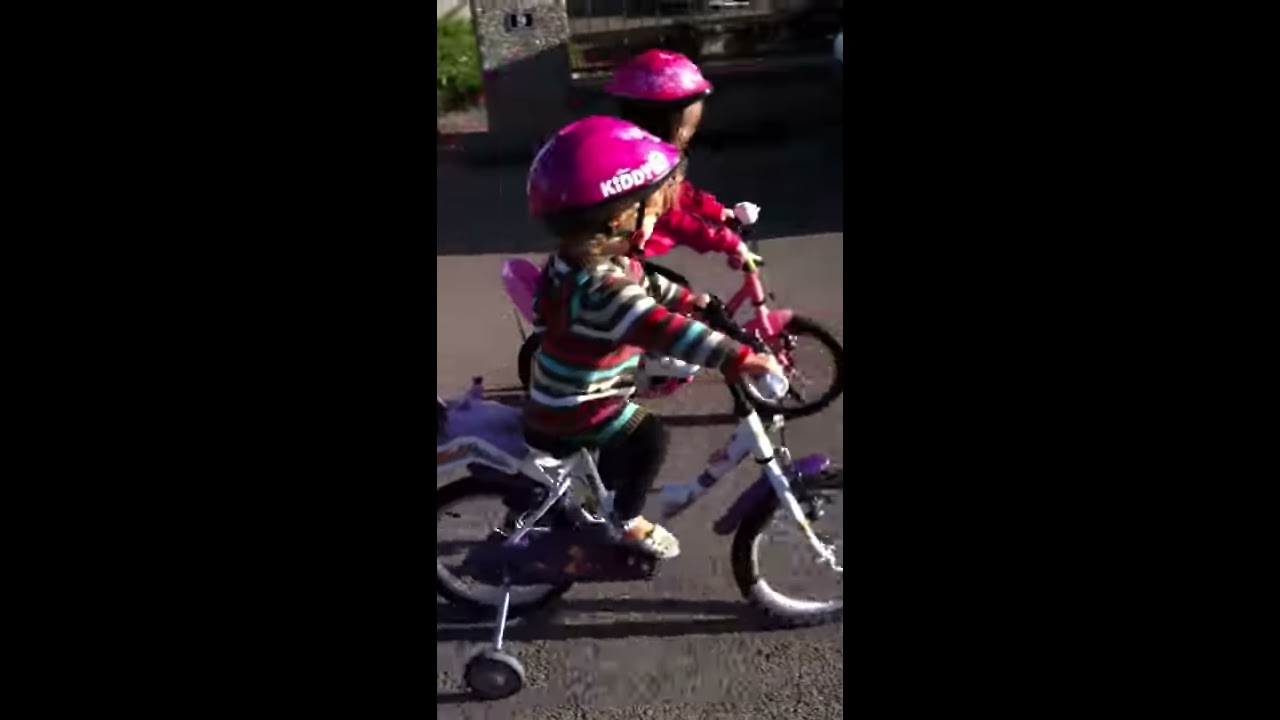In this image, we see two young girls riding bicycles with training wheels on an asphalt road. Both girls are wearing long-sleeved clothing and pink helmets, potentially labeled with the word "Kitty." The girl closest to the front and center of the image is on a white-framed bicycle with purple fenders, dressed in black pants, white shoes, and a striped shirt featuring red, white, black, and teal colors. Beside her, slightly behind, the second girl rides an all-pink bicycle and wears a red shirt. The scene is set outdoors in the middle of the day, with a distant building and trees visible in the top left of the image. The colors in this photo include grey, white, black, purple, pink, light blue, red, and green. The image quality is described as low resolution, and some black framing is present on the left and right sides.